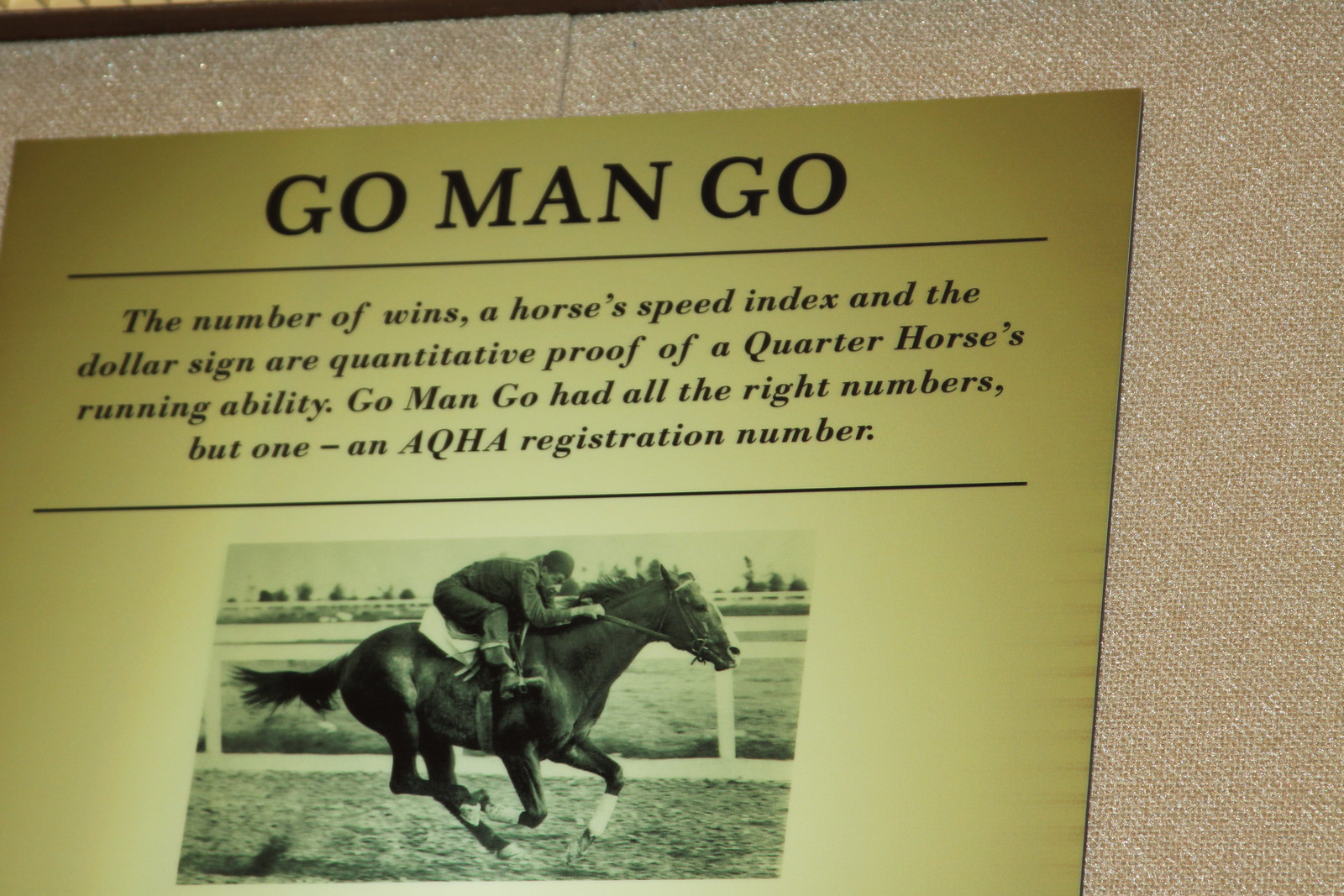The image features an informational sign pinned to a fabric-covered bulletin board. At the top of the sign, "GO MAN GO" is prominently displayed in all capital letters. Below this bold heading, an italicized inscription reads: "The number of wins, a horse's speed index, and the dollar sign are quantitative proof of a quarter horse's running ability. GO MAN GO had all the right numbers but one, an AQHA registration number." This text highlights the essential statistics that reflect a quarter horse’s performance and specifically points out the missing American Quarter Horse Association registration number for the horse named "GO MAN GO." Beneath the text, there is a black-and-white, side-profile photograph of a jockey riding a mid-gallop, brown horse, racing towards the right-hand side of the image. The sign, printed on thick stock paper, appears to be carefully positioned on a typical bulletin board suitable for pinning notices and announcements.